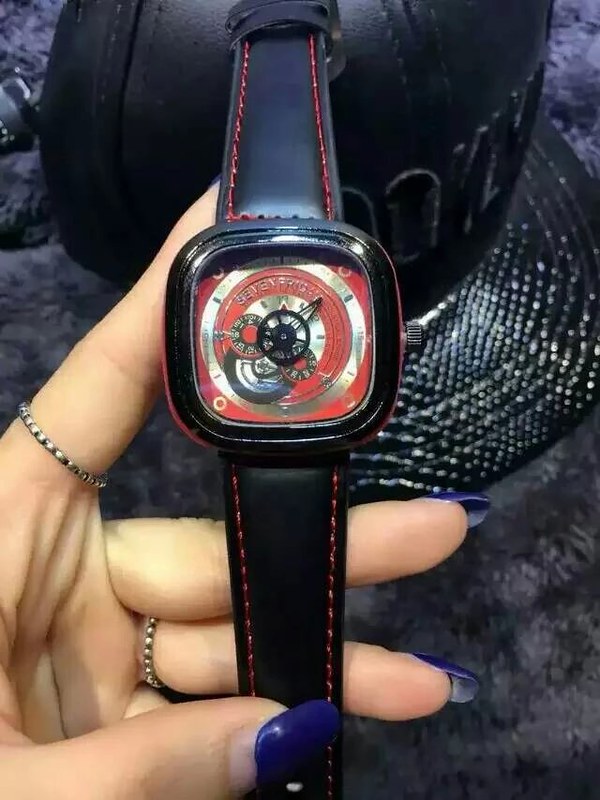In this detailed image, a woman's left hand is prominently centered, holding a striking watch. Her fingernails are long, artificial, and painted a dark navy blue, extending slightly beyond the midpoint of her natural nails. On her pale-skinned hand, she wears two thin, grooved metal rings, one on her index finger and the other on her ring finger.

The watch itself is the focal point of the photograph. It boasts a sleek black leather strap with meticulous red stitching running down both sides. The watch's rectangular face with rounded edges displays a mesmerizing red and silver spiral pattern, with visible gears at its center. Instead of traditional numbers, the face is marked only at four equidistant points, enclosed by a silver band, and surrounded by a black housing.

In the background, the image features a black baseball cap adorned with sparkling gems and raised letters, though the text is indistinct. The cap's reflective bill catches and scatters light, revealing gray dots. A soft, plush blanket with a velvety texture envelops the scene, further adding to the cozy ambiance.